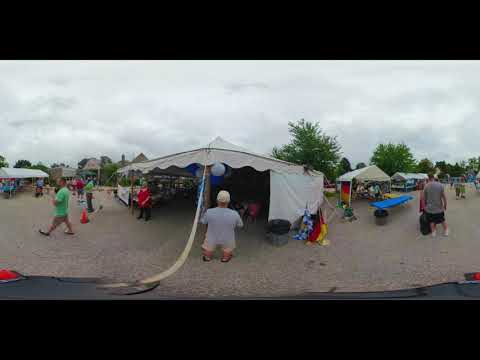The photograph captures a bustling outdoor festival set on a spacious dirt or concrete-like ground. Central to the scene is a large white circus-style tent with openings on two sides. Blue balloons adorn the top of this tent, adding a touch of vibrancy. A man stands in front of the tent with his back to the camera, dressed in a light blue shirt and white hat. Scattered around are multiple other white tents, where people are selling various goods and offering services.

The festival appears to be quite crowded, with numerous individuals clad in summer attire — shorts and short-sleeved shirts — indicative of the warm, albeit overcast day. On the left side of the image, a man in a green t-shirt, khaki shorts, and sandals is visible. On the right, next to a blue bench, stands another man wearing a gray shirt and black shorts. Front and center, under the main tent, is a woman in a red short-sleeved shirt and black trousers.

The sky is cloud-laden, casting a gray hue over the festivities, while dark green trees in the background provide a natural frame to the scene. The overall atmosphere suggests a lively, community-oriented county fair with an array of attractions, potentially including carnival games and other entertainment.